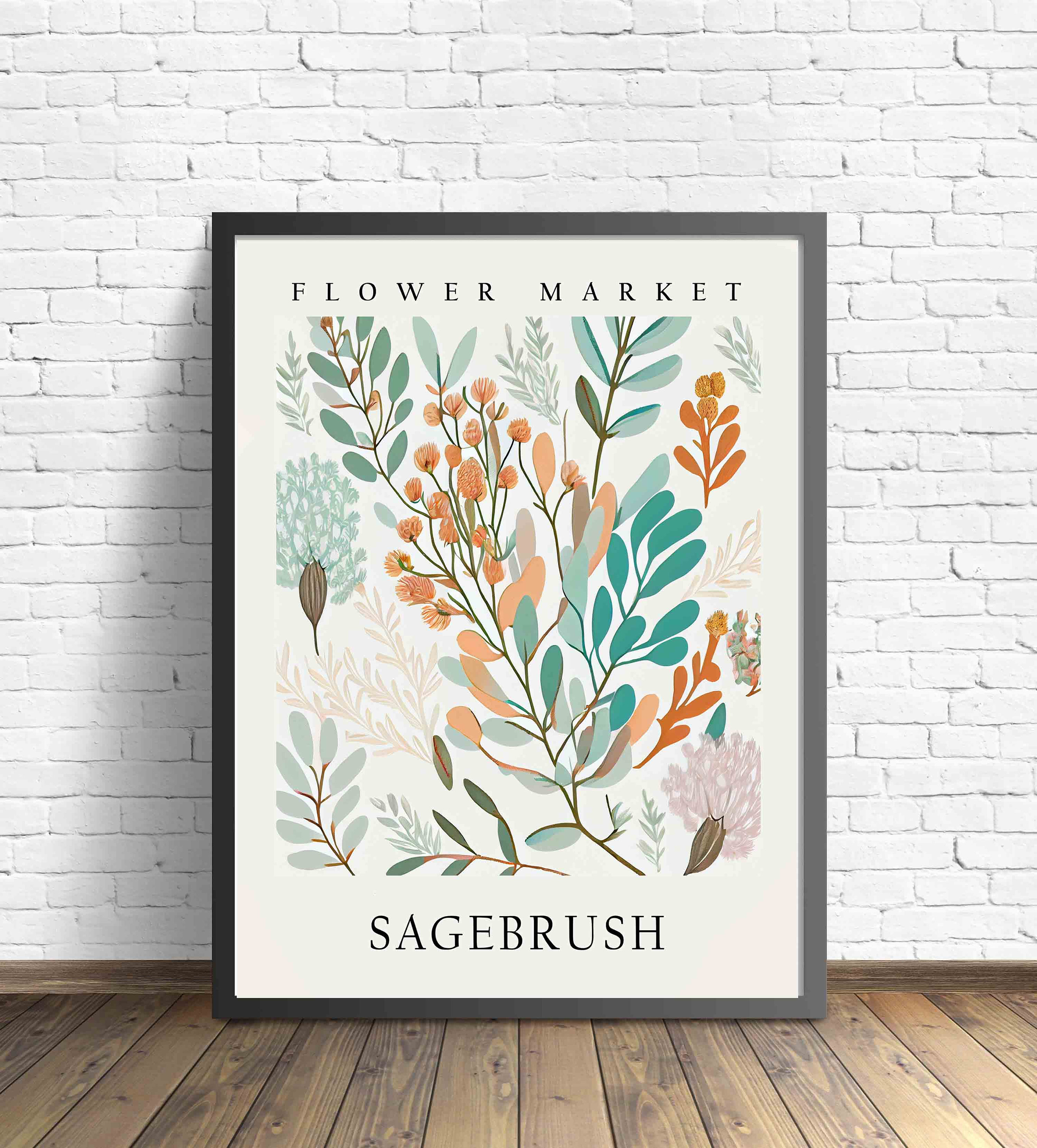The image depicts a blackish-gray framed piece of wall art leaning against a white-painted brick wall. The floor beneath it consists of vertically aligned wooden planks. The frame encloses a white background that features the text "Flower Market" at the top and "Sage Brush" at the bottom, both in black font. The artwork showcases an assortment of flowers and plants, including green, orange, and pinkish flowers in vibrant hues, as well as leaves in varying shades of green, yellow, and red. Some of the plants in the illustration are more vibrant, while others appear more faded, adding depth to the composition. Additionally, there are what appear to be fruits on the left side and the bottom right corner of the artwork.